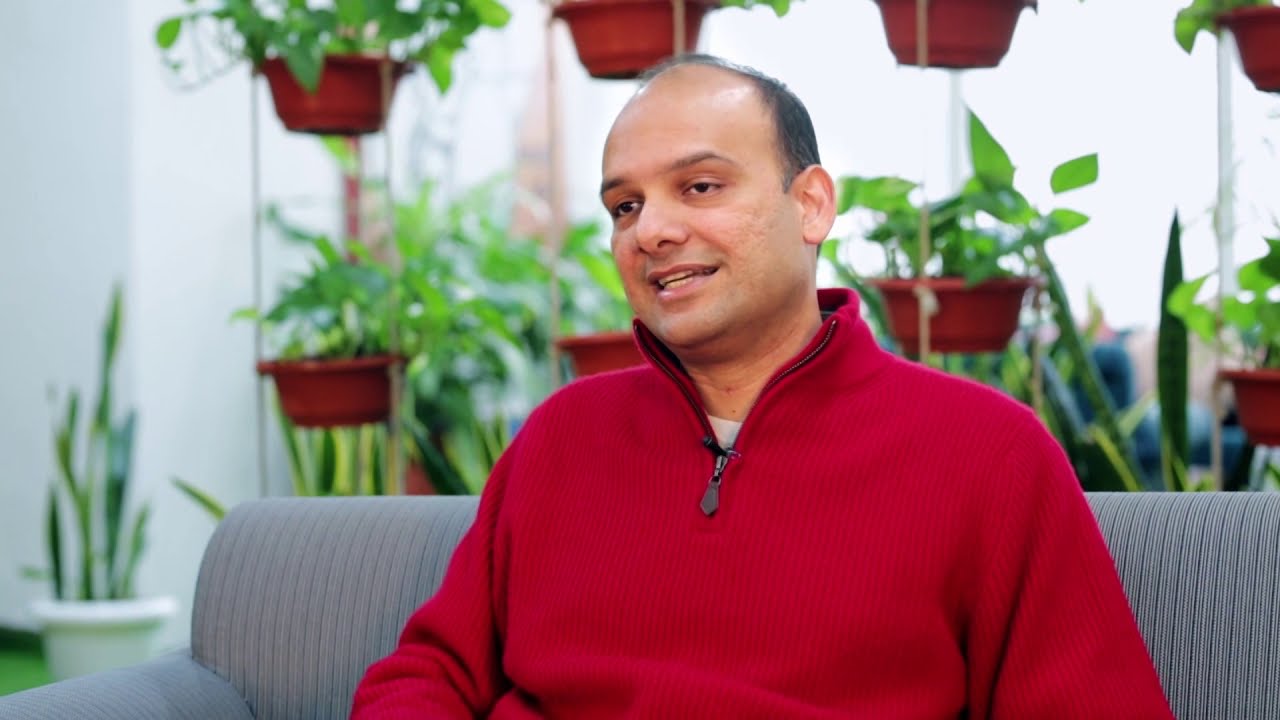In a brightly lit indoor setting, a man sits on a grey, striped couch positioned centrally in the image. He is clothed in a red long-sleeved sweater, partially unzipped from his leg to his upper chest, revealing a microphone attached to his collar—suggesting he might be in the midst of an interview. The man is looking off to the left side with a visible smile that displays the lower rows of his teeth. The background features a white wall adorned with numerous green plants in various potted arrangements. Some plants are suspended from the ceiling, while others are placed on shelves or sit on the floor, enhancing the natural ambiance of the space. Visible through what seems like a large glass window, ample daylight floods the room, highlighting the array of white, green, gray, red, tan, and brown colors throughout the scene. A white planter with long green plants also appears at the bottom left corner, adding to the lush greenery.